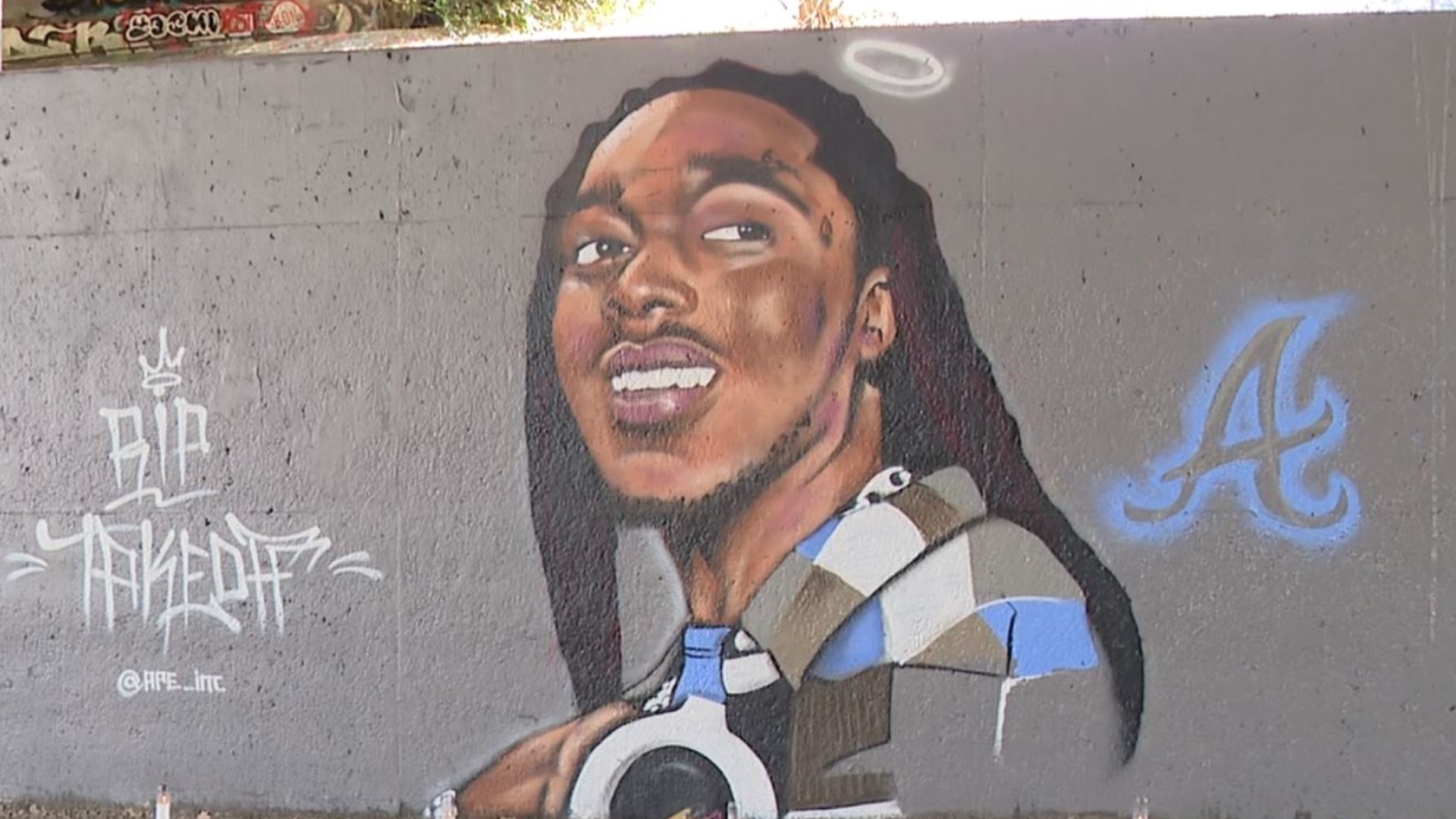The photograph captures a vibrant graffiti-style mural painted on an otherwise grey wall. Central to the artwork is the image of a smiling man with black skin and long black hair. He stands out in his geometric-style top adorned with a pattern of white, grey, and blue squares. Adding a somber yet respectful tone to the mural is a graffiti tag reading "RIP Take Off" situated next to the man. On the opposite side, a bold blue letter 'A' punctuates the scene. Above the man's head, a delicate halo ring floats, adding an ethereal touch to his depiction.